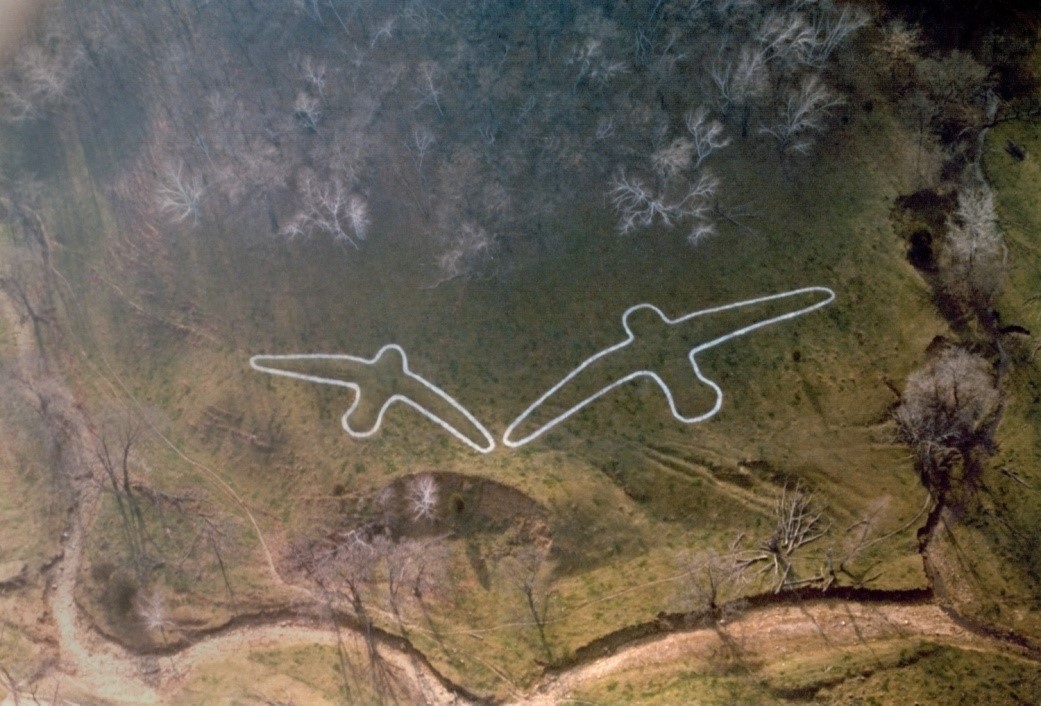This is a color aerial photograph in landscape orientation, capturing a large grassy field bordered by a dry riverbed at the bottom and a stand of dead trees near the top center. At the core of the image, two white outlined birds in flight are clearly depicted, each with wings outstretched, angled toward each other. These outlines appear to be painted directly on the grass or possibly digitally added to the photograph. The scene suggests a secluded meadow nestled in a wooded area, enhancing the serene, natural composition of the field. Sparse, spotty trees flank the sides of the image, with mounded dirt sections visible along the bottom, adding depth and detail to the expansive outdoor setting.